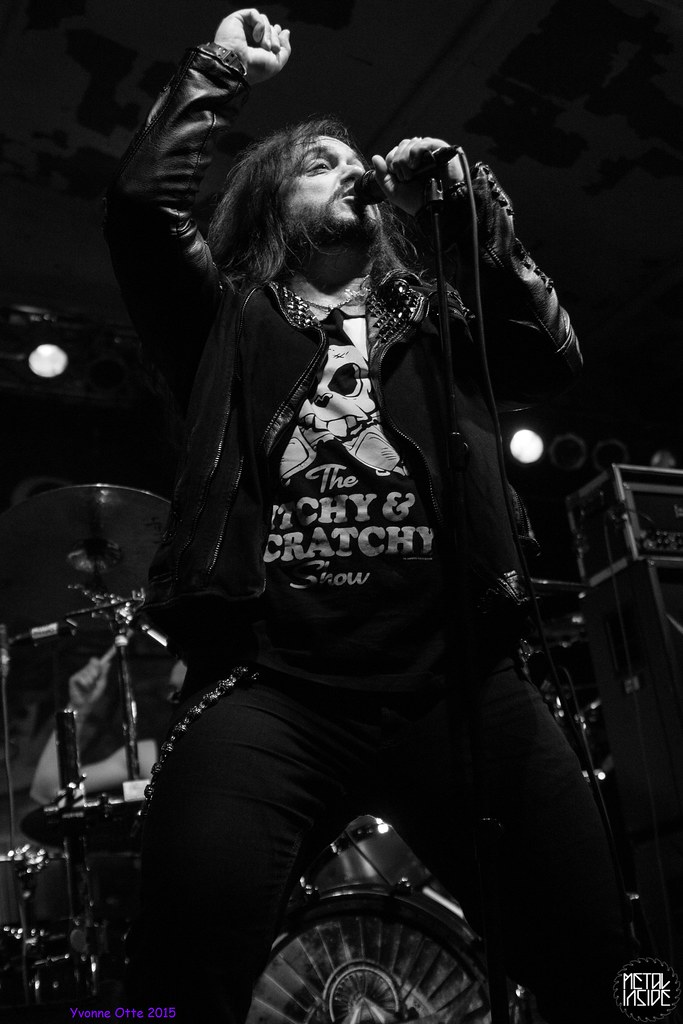The image is a black-and-white photograph capturing a dynamic moment of a man performing on stage, inferred by the low-angle perspective that shows him from his knees upwards. He sports tight black denim pants, featuring a distinctive chain running from the belt loop down and looping back up on his right leg. His attire includes a black graphic T-shirt adorned with a large skull and white text reading "The Itchy and Scratchy Show," partially obscured by a black leather jacket with studded collars. The man, who has long dark hair, a beard, and a mustache, grips a microphone pointed towards his face, attached to a stand, while his other hand is raised in the air, capturing his energetic stage presence. Behind him, a drum set and an amplifier can be partially seen, with a person poised to strike the drums with a light brown drumstick, adding to the concert ambiance.